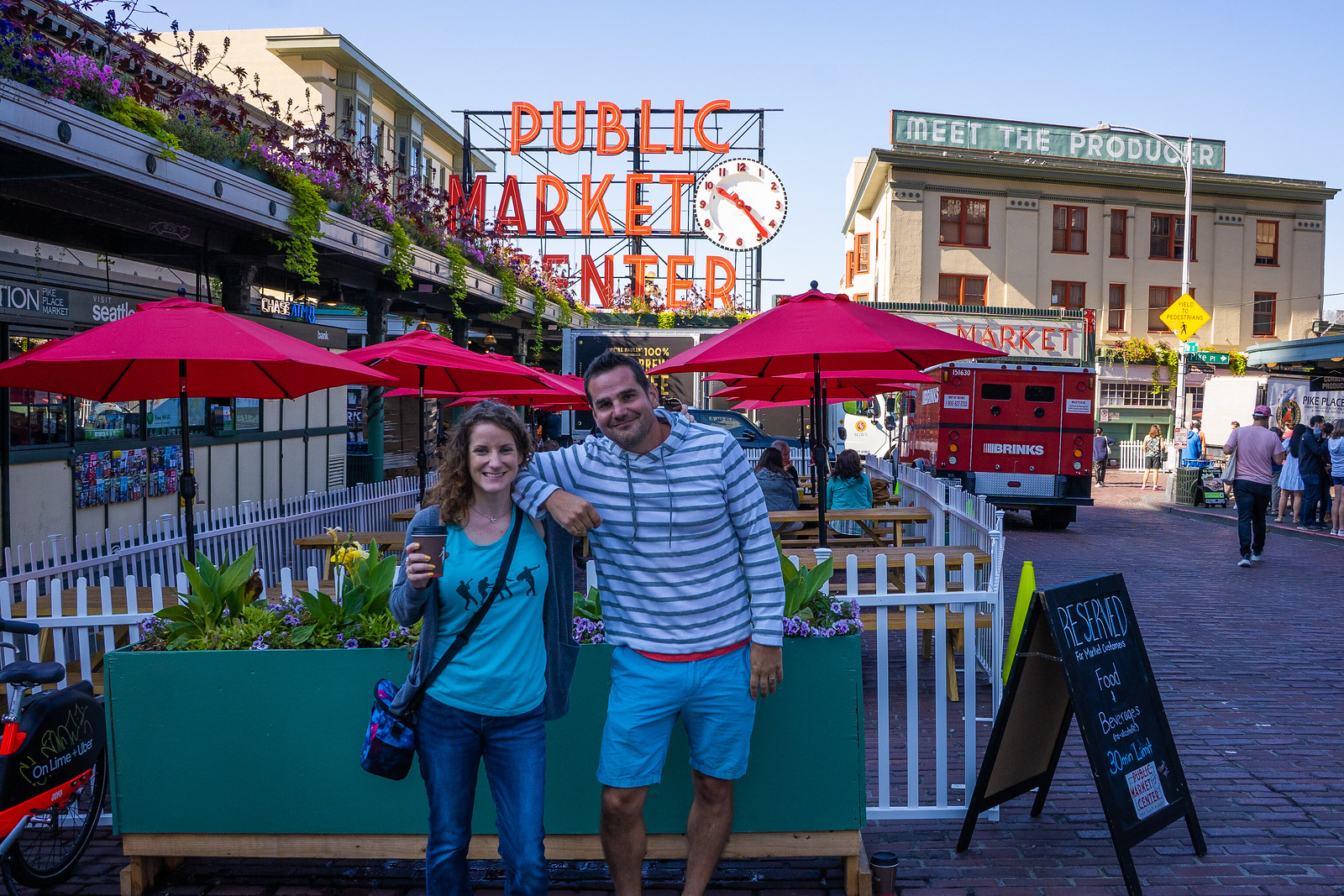In this vibrant, clear-skied photograph of Portland, Oregon's iconic Public Market Center, two smiling young individuals are the focal point, standing side by side in front of a bustling market square. The man, casually dressed in a white and blue striped long-sleeve hoodie and light blue shorts, has his arm comfortably resting on the shoulder of the woman beside him. She is wearing an aqua t-shirt, dark blue jeans, and a black shoulder bag. Both are looking directly at the camera, their expressions filled with cheer.

The background showcases the market's renowned red neon sign proclaiming "Public Market Center," complete with a white clock displaying the time as 4:50. The scene captures the essence of a lively market day, with a backdrop that includes a beige two-story building adorned with a green banner reading "Meet the Producer," and bordered in red window frames. A red truck, bearing a resemblance to a Brinks vehicle, is parked on the brick-paved street to the right, adding a dash of colorful urban activity.

Adding to the ambiance, a fenced dining area with white picket fencing and red umbrellas over wooden benches sits behind the pair, filled with patrons enjoying the day. The brick road to the right is busy with other market-goers, enhancing the bustling, community atmosphere of this picturesque farmer's market setting. The photograph captures a moment of urban vitality and charm, framed with natural flowers on the left and brightly colored signs that celebrate the local flair.